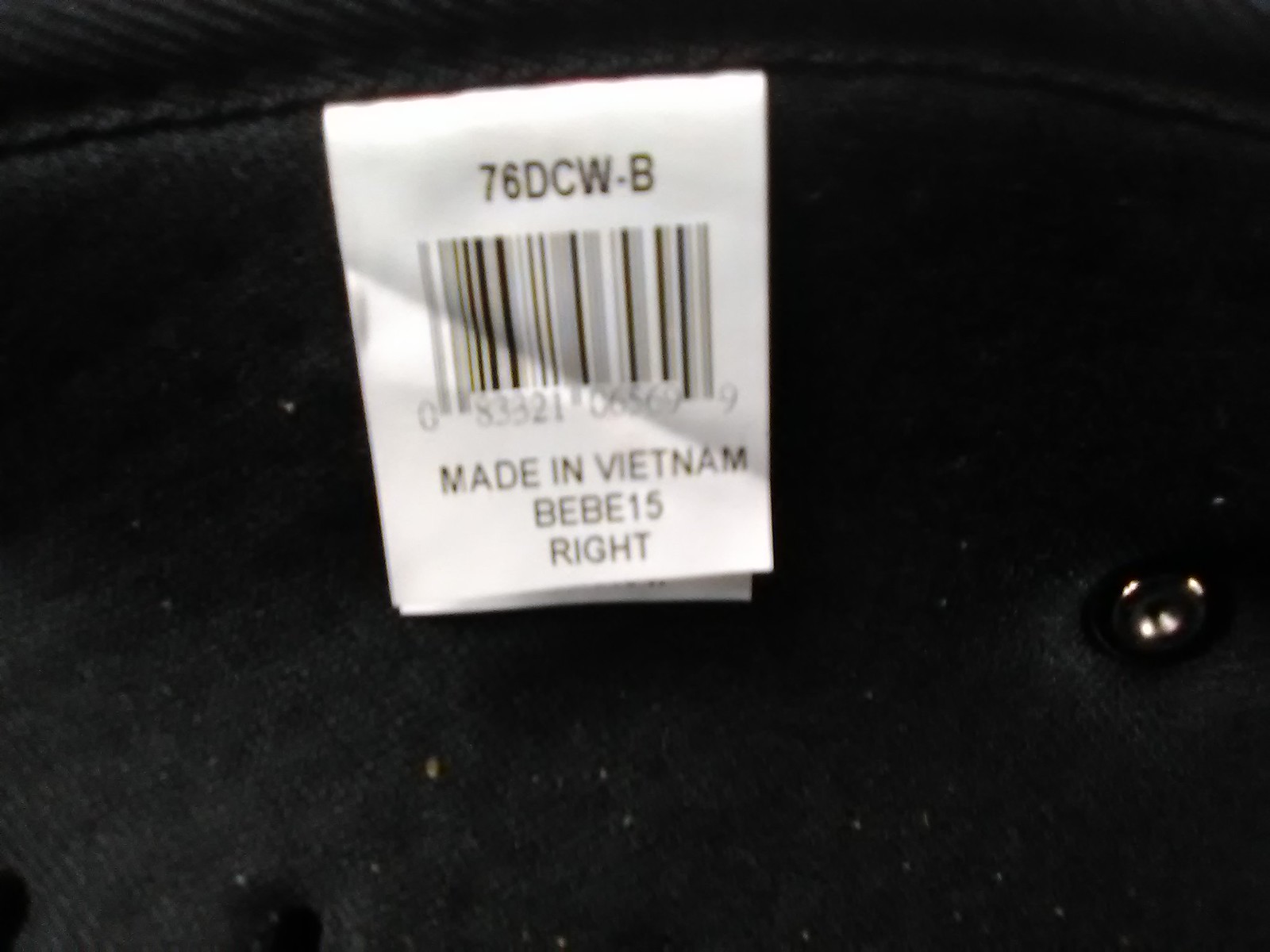The up-close image features a white tag affixed to a textured, velvety black surface, possibly the fabric of a chair or a piece of clothing. The tag prominently displays the code "76DCW-B" at the top in black letters. Directly beneath this code is a barcode, with the numbers "08332106569" in a small font along the top edge. Below the barcode is the text "Made in Vietnam," followed by "BEBE15" and "Right" (spelled out as "R-I-G-H-T"). To the right of the tag, there appears to be a shiny black button, while the bottom left of the image displays what could be two buttonholes, accentuating the complex, stitched detailing. Further inspection suggests another tag may be underneath the visible one, adding to the layered complexity of the scene.